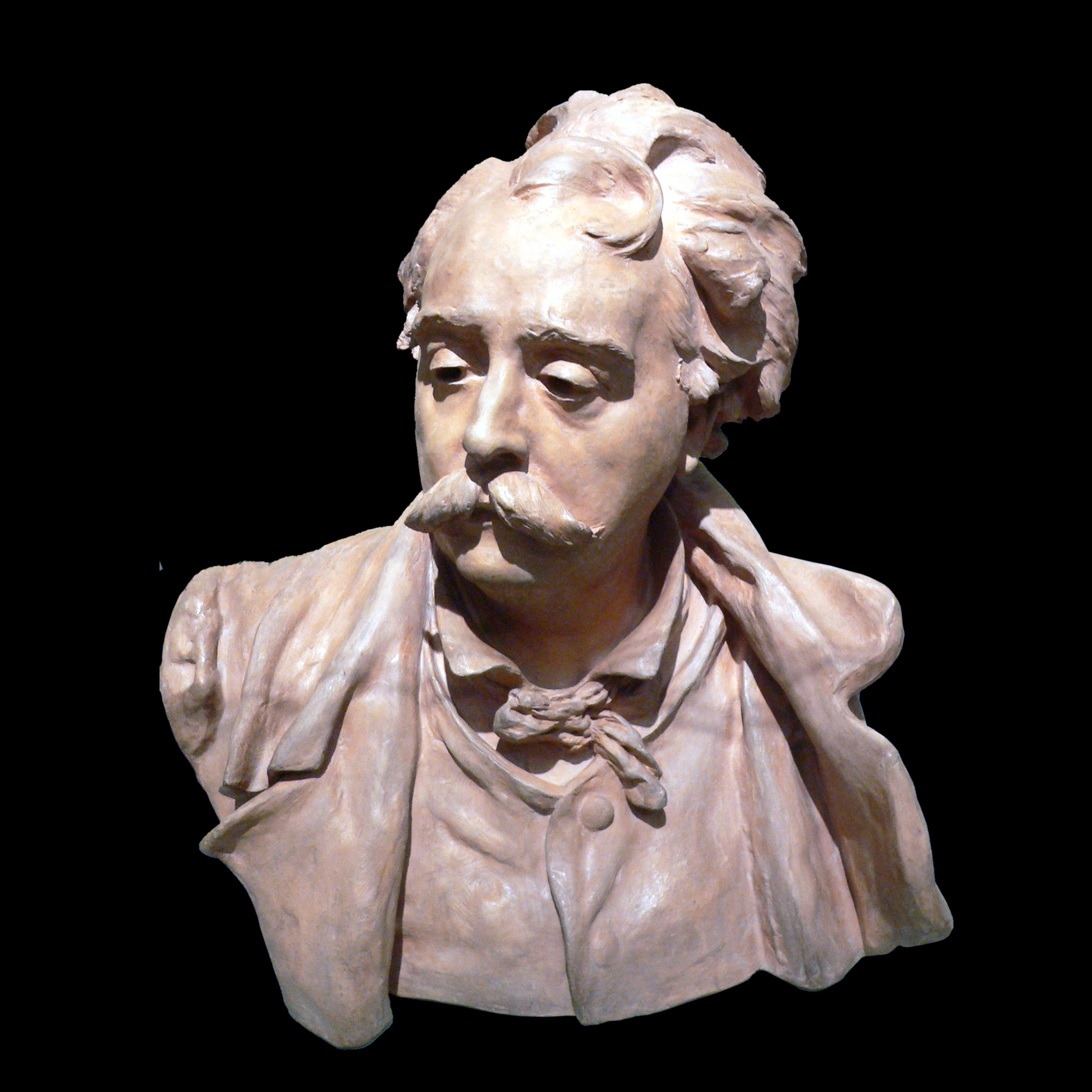The image features a detailed clay bust of an elderly man, portraying him from the middle of the chest to the top of his head. The bust, crafted from a mixture of darker browns and oranges, is set against a flat black backdrop, giving it the illusion of floating. The man has a prominent mustache, a high forehead with a central curl in his otherwise looped back curly hair, and heavy eyelids casting shadows over his downcast eyes. His face, characterized by a straight nose with thin nostrils, is turned slightly down towards the left. Dressed in an old-fashioned outfit, he wears a collared shirt with a tie, over which a button-up vest and jacket are layered. The lighting accentuates the textures and shadows, adding depth to the facial features and the intricacies of the clothing.